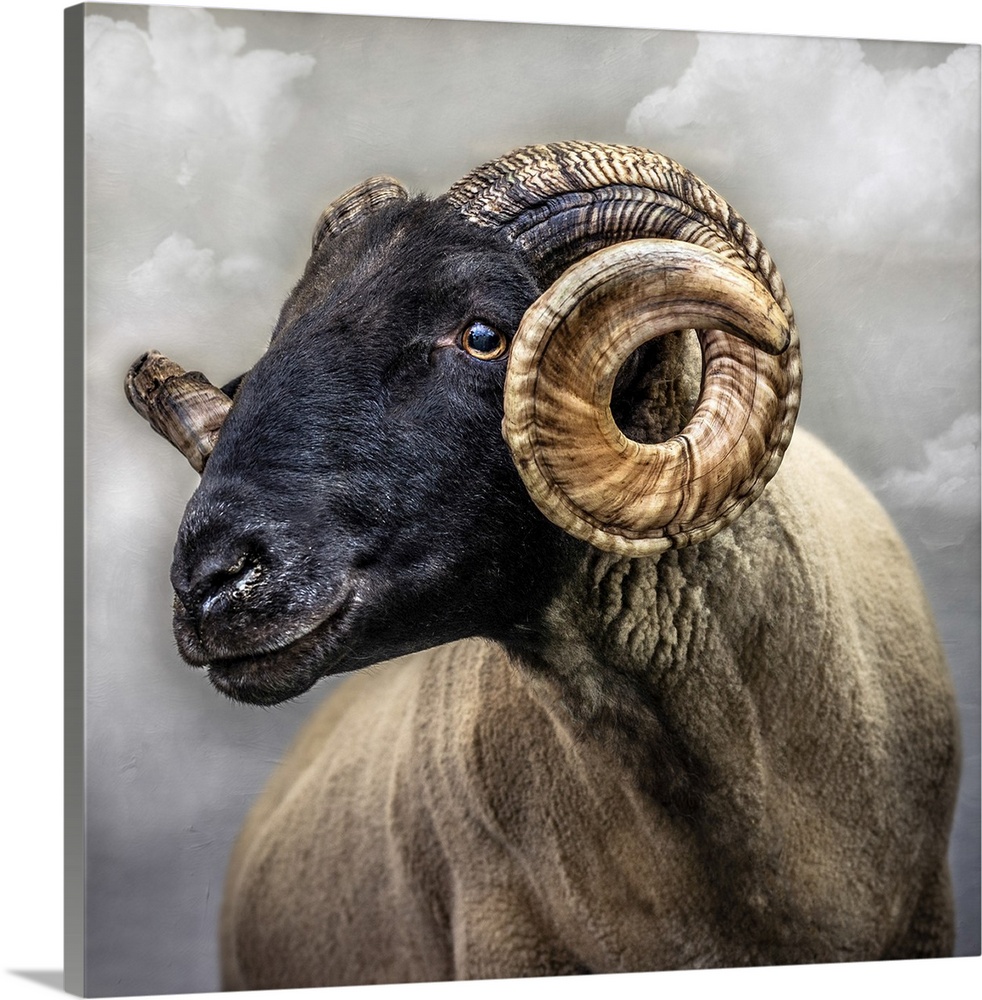The image showcases a highly detailed painting of a ram, presented in a rectangular, horizontally-aligned canvas with a visible gray-painted edge, casting a soft shadow on a plain white background. The ram's body, predominantly tan with a slight wave pattern in its fur, occupies the right center of the composition. Its head, which is mostly black, angles back towards the left, forming a rough V-shape with its body. The ram has impressively large, curled horns: tan at the base with black stripes and notches, and they curve in an oval shape rising from the head. The horns' intricate detailing, resembling a mix of scales and grooves, adds to their realism. The ram's eye features a yellow iris and a black pupil, standing out against its dark fur. The background consists of a cloudy gray sky with well-defined patches of white and gray clouds, enhancing the ram's striking appearance. The painting is a meticulous depiction, capturing every hair and subtle reflection in the ram's eye, almost appearing as if the animal could step out of the canvas.